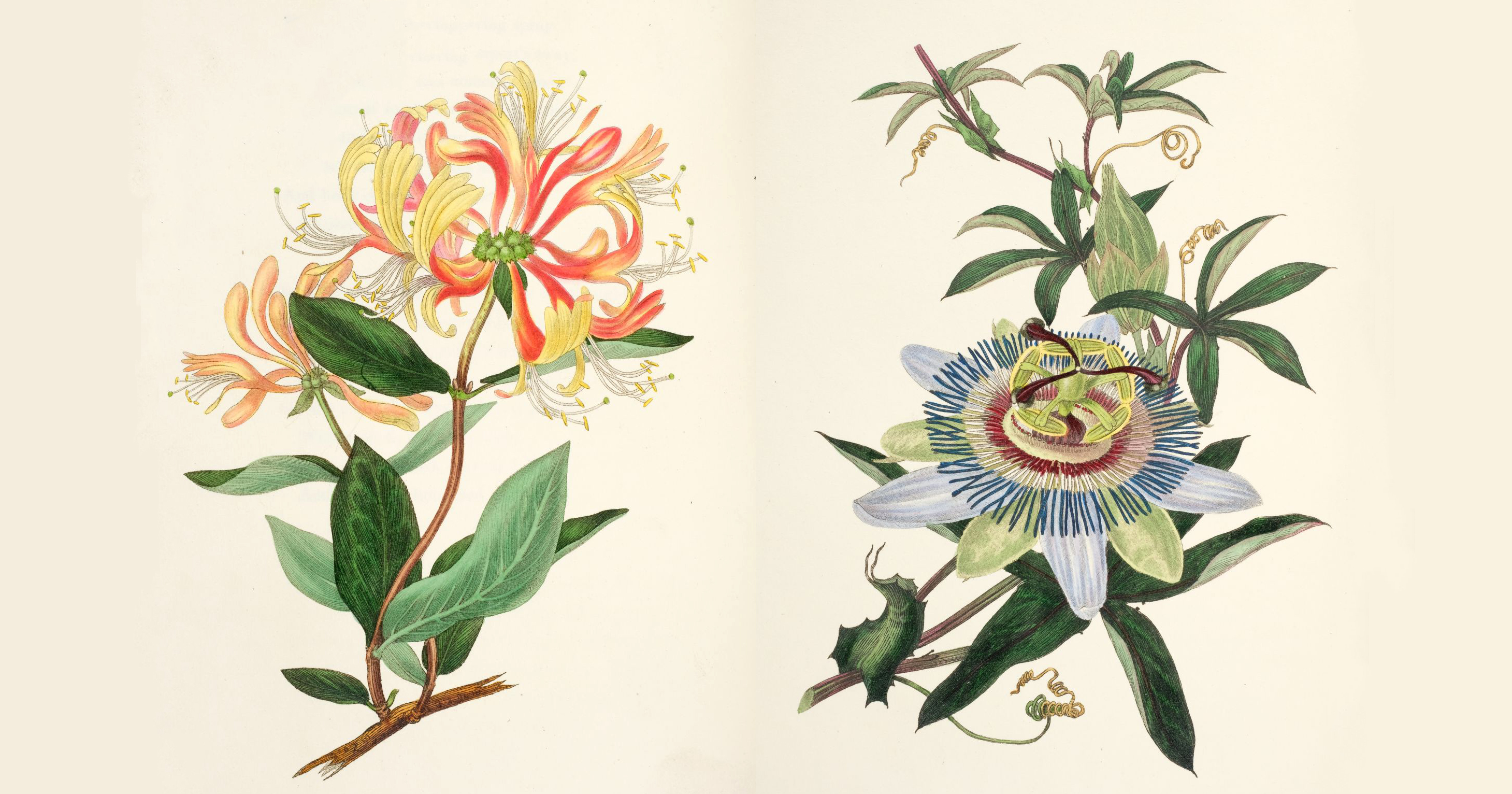The image presents two hand-sketched or painted floral elements side by side, set against a light tan ivory background. Both flowers are centrally placed, equally occupying the left and right halves of the image, which is horizontally oriented. The left flower showcases a reddish-yellow bloom with green leaves at the base, characterized by long green stems. The petals exhibit corally hues transitioning to yellow at the tips, surrounding a green center. In contrast, the right flower resembles a sunflower, featuring petals that alternate between light blue and light green, with a dark purple-red center. The leaves are similarly green, but with alternating dark and light shades, supported by a brown stem. The image is void of any textual elements or artist signature, emphasizing the intricate, high-quality details of the floral illustrations.